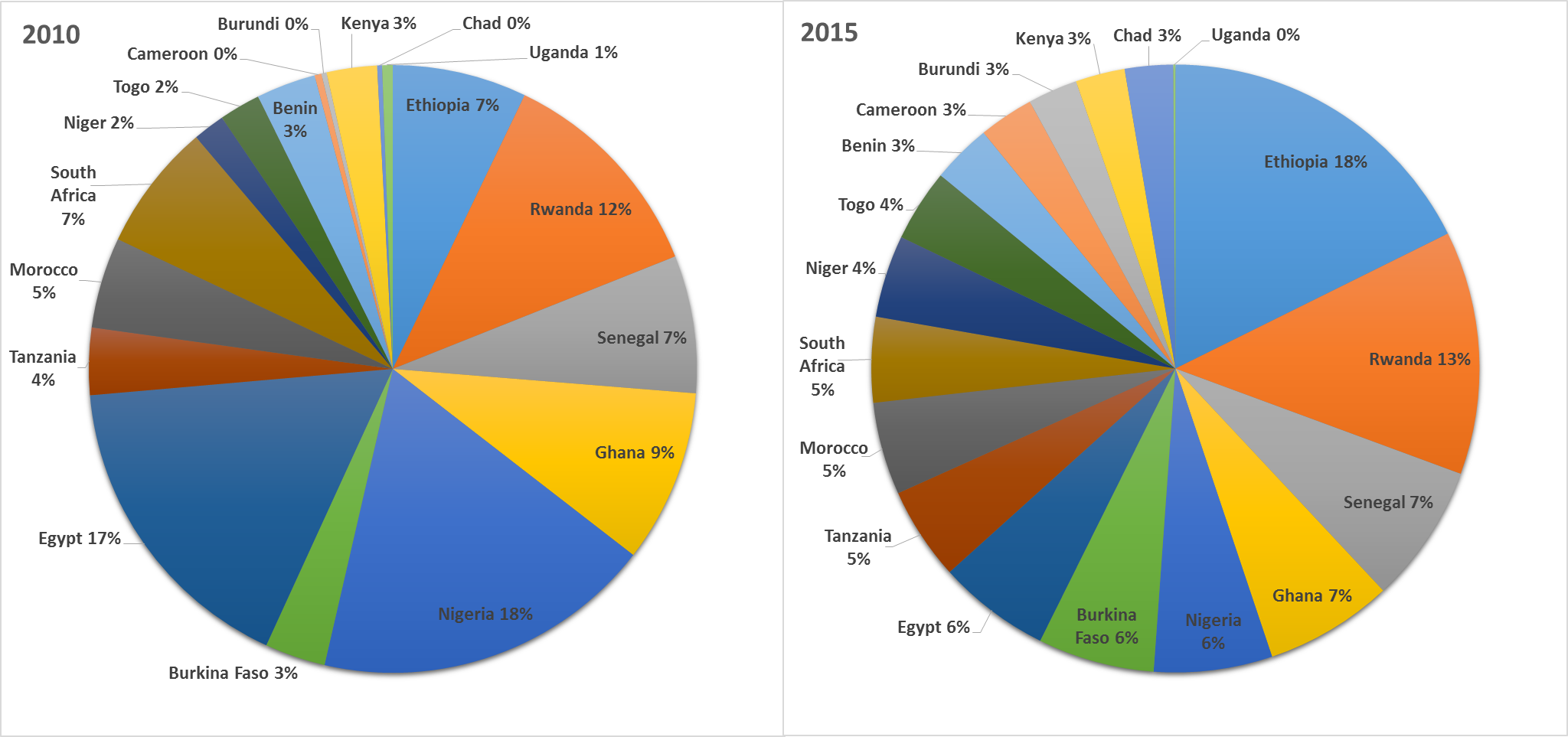The image showcases two pie charts side by side, with the left chart representing data from 2010 and the right chart representing data from 2015. Both pie charts are labeled with the names of various African countries: Burundi, Kenya, Chad, Uganda, Ethiopia, Rwanda, Senegal, Ghana, Nigeria, Burkina Faso, Egypt, Tanzania, Morocco, South Africa, Niger, Togo, Cameroon, and Benin. The left chart for 2010 shows the largest portions occupied by Egypt and Nigeria, with Nigeria making up 18%. The right chart for 2015, however, indicates a shift, with Ethiopia and Rwanda becoming the largest segments, with Ethiopia comprising 18%. Each segment of the charts is color-coded but lacks a legend explaining the colors. The charts appear to be intended for educational or analytical purposes, set against a plain white background to emphasize the data.